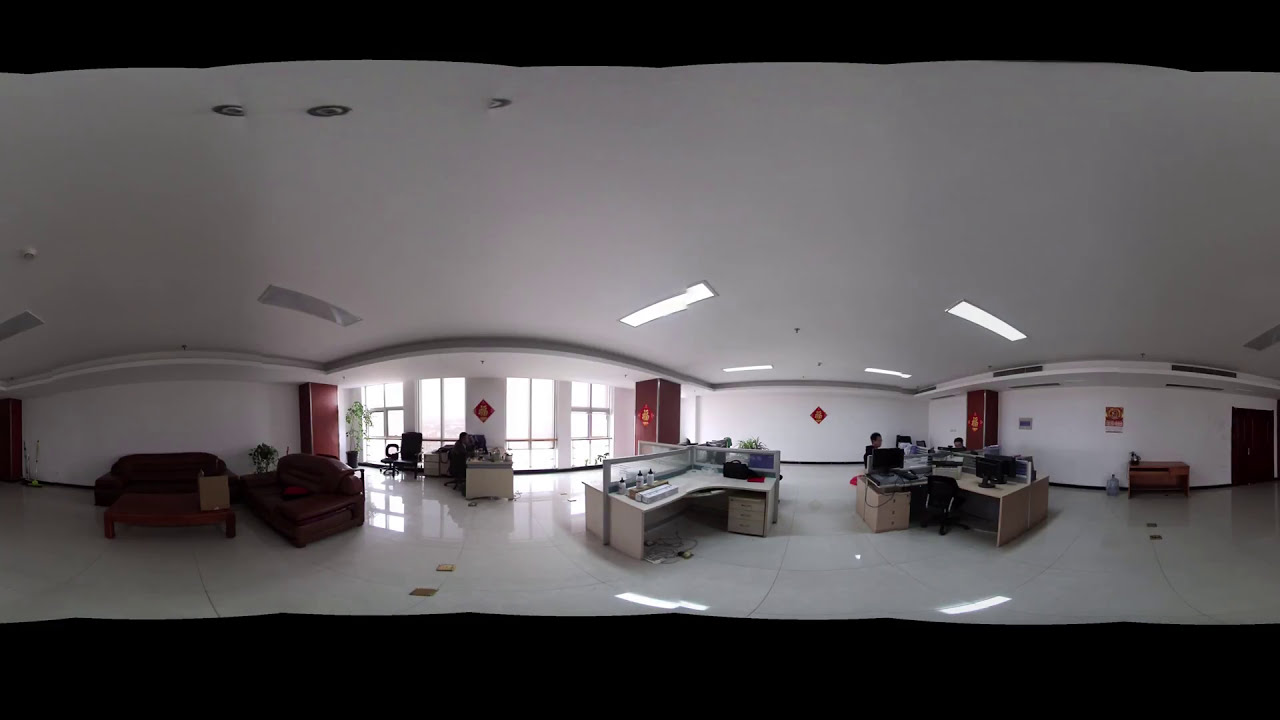This image portrays an expansive, sparsely furnished office space with a minimalist, startup vibe. The room is predominantly white, featuring white floors, walls, and ceilings illuminated by fluorescent lights and accompanied by silver ceiling vents. The walls are intermittently adorned with reddish posts and red-and-white diamond-shaped signs. 

In the center of the space sit several desks, equipped with multiple computer monitors, suggesting a highly functional yet minimalistic work setting. The focal point includes a total of four desk spaces, with two of them occupied by people working. On the right-hand side, a small group is gathered around a desk. Near the center, between two prominent windows, there is either another desk or a cart.

The office also contains a cozy break area to the left, furnished with brown or black leather couches and a small coffee table. To add a touch of greenery, a couple of ficus trees and plants in black flower pots are situated strategically around the room. The overall aesthetic suggests a recently established office, just getting started with its essential furniture and equipment. The large room, with its few pieces of furniture, projects a sense of openness and potential.